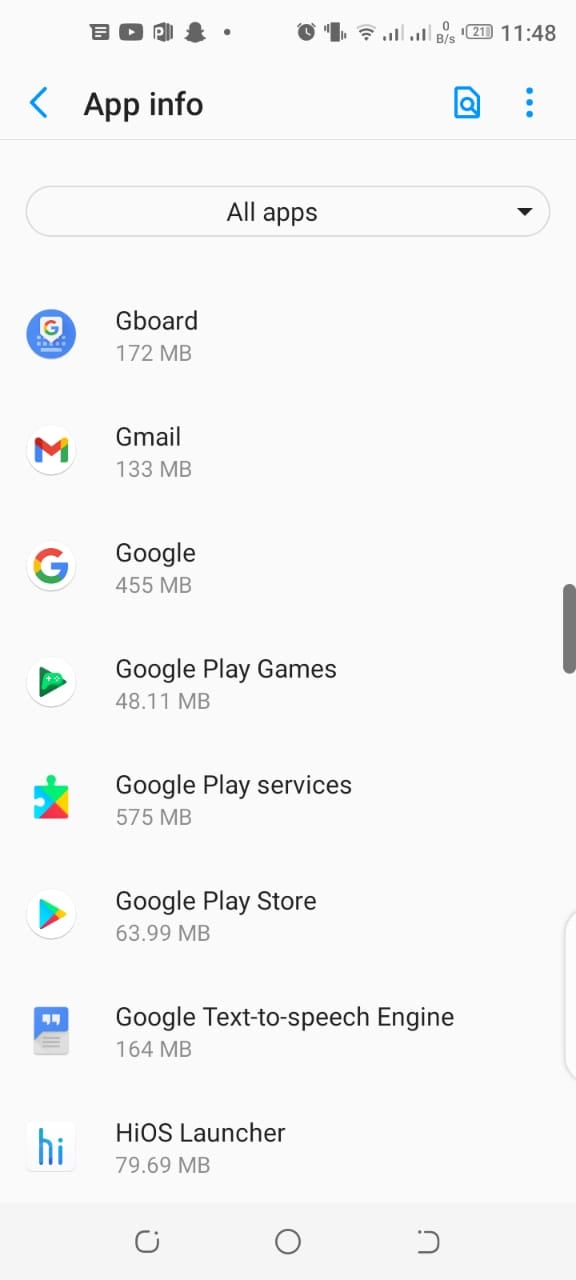The image depicts the screen of a smartphone displaying the "App Info" section. The screen shows various metrics and details about the apps installed on the device. At the top, in black text, is the label "App Info," with a blue left arrow, a vertical three-dot menu icon, and a magnifying glass icon symbolizing search functionality. 

Below this, there's a drop-down menu labeled "All apps." The list includes:
- Gboard: 172 MB
- Gmail: 133 MB
- Google: 1,455 MB
- Google Play Games: 48.11 MB
- Google Play Services: 575 MB
- Google Play Store: 63.99 MB
- Google Text-to-Speech Engine: 164 MB
- HIOS Launcher: 79.69 MB

The screen also shows standard status indicators: the YouTube icon, current time (11:48), battery level (21% charge), vibration mode, Wi-Fi status, and signal strength bars. At the bottom of the screen are the navigation tools, represented as a broken circle (perhaps Back or Recent Apps), a full circle (Home), and a half-circle (possibly an Overview or Menu button).

The overall color scheme predominantly features blue, red, yellow, and green, which are commonly associated with Google app icons. The detailed breakdown of storage usage highlights how much memory each individual app occupies on the device.